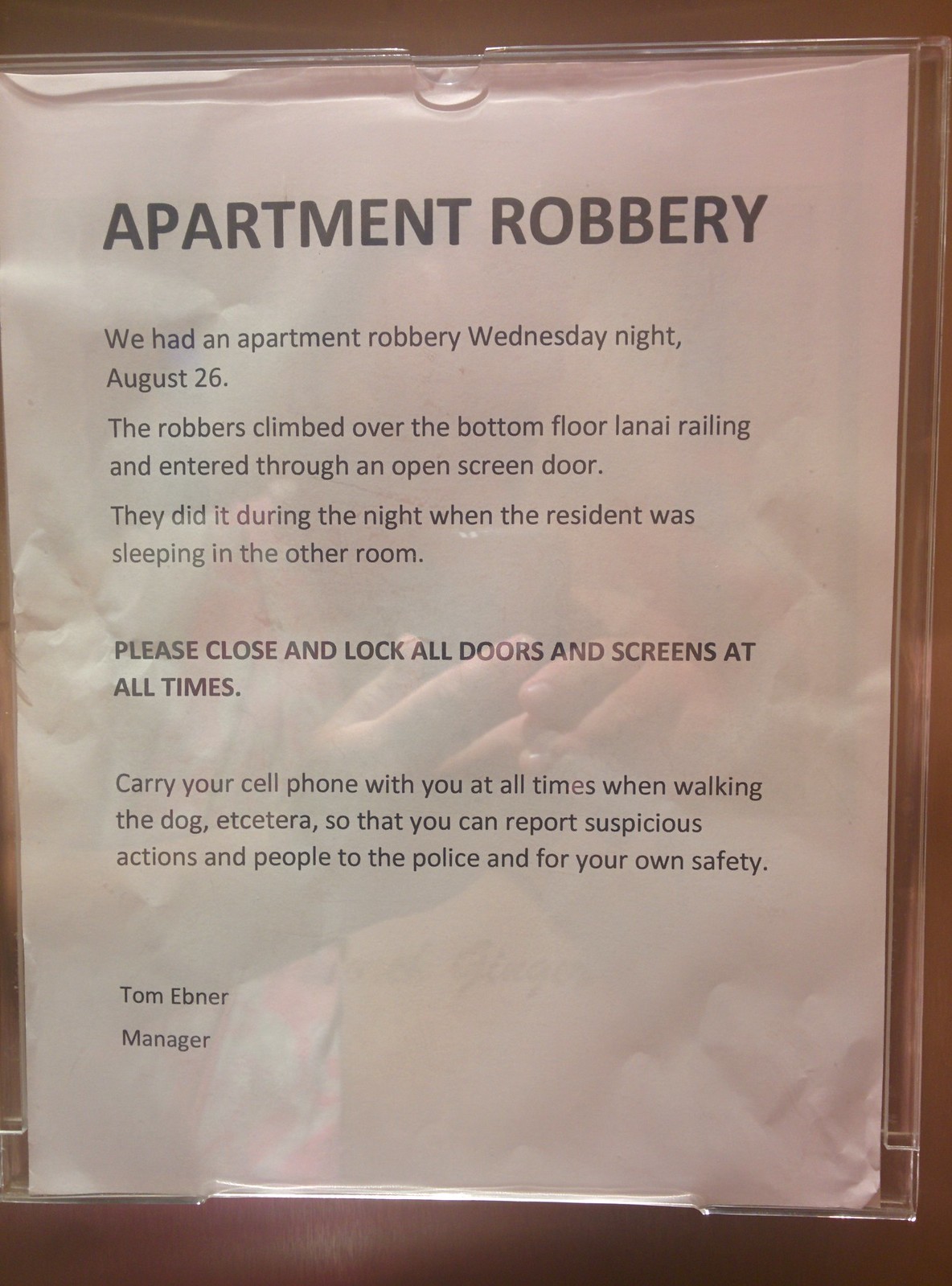The image displays a white rectangular sign posted on a brown wall, enclosed in a clear plastic frame. At the top, in bold black letters, it announces "Apartment Robbery." The sign details that an apartment robbery occurred on Wednesday night, August 26. The robbers accessed the apartment by climbing over the bottom floor lanai railing and entering through an open screen door while the resident was asleep in another room. In bold letters, it advises, "Please close and lock all doors and screens at all times." Below that, it includes a reminder to "Carry your cell phone with you at all times when walking the dog, etc., to report suspicious actions and people to the police for your own safety." The notice is signed at the bottom by Tom Ebner, the manager.